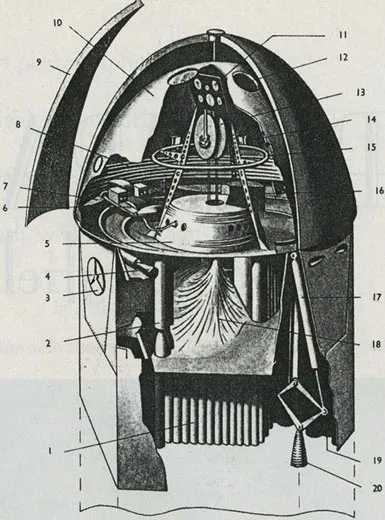The black-and-white image showcases a detailed cross-section diagram of a complex, dome-shaped mechanism, revealing its intricate inner machinery. The device is methodically labeled with numbers ranging from 1 to 20, each pointing to specific components, but without accompanying descriptions. The diagram appears to be divided into two levels, intricately packed with various long and round parts. On the top center, there's a discernible pulley system intertwined with ringed wires that likely contribute to its functionality. The bottom part of the device exposes several tubes connected to a larger set of tubes on the ground, and a wire apparatus situated on the right side. The numbering system is divided, with 1 through 10 on the left side in ascending order and 11 through 20 on the right side descending from top to bottom. The overall backdrop of the image is light gray, enhancing the visibility of the dark-colored components within the device. Despite the detailed visual depiction, the exact function of the mechanism remains unidentified.